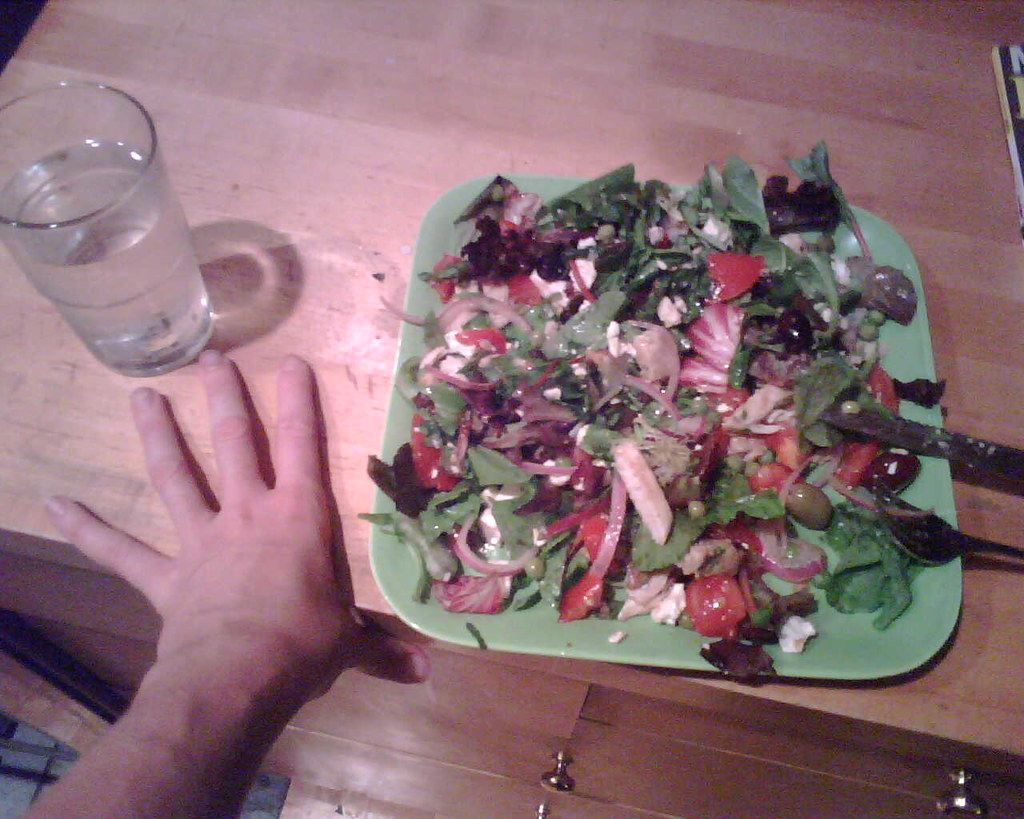This is a photograph looking down at a light, butcher block style wooden table with muted colors, giving it a slightly grainy texture. On the bottom left corner, a left hand is visible with four fingers splayed on the tabletop and the thumb resting on the side. Just above the hand, there is a three-quarters full clear glass of water casting a circular shadow next to it. Centered on the table is a square plate with rounded edges in a pale green color, holding a vibrant, colorful salad. The salad is a generous mix of fresh greens including lettuce and purple cabbage, complemented by sliced red onions, juicy tomatoes, black olives, and sprinkled bits of feta cheese. A knife and fork are positioned at the sides of the plate, ready for use. Golden knobs from a drawer or cabinet below the table can also be seen on the front, adding a touch of detail to the scene.